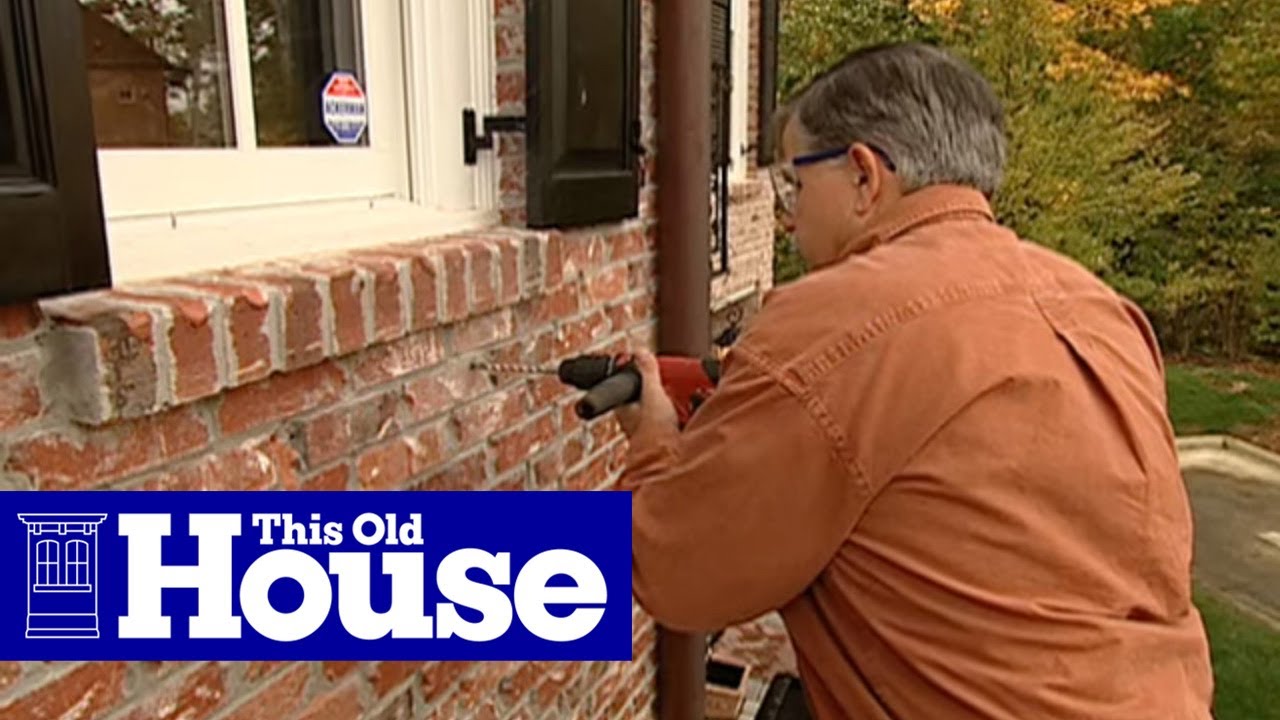A detailed horizontal rectangular photograph captures a man in his 40s or 50s, dressed in an orange shirt and safety glasses, working outdoors during the daytime. The man, who has short graying hair, is seen in profile though his back is mostly turned to the camera, is using a red and black power drill to drill holes into a well-worn red brick wall. Above the brick wall is a window ledge with a white frame and black shutters, along with an unfocused red, white, and blue security sign. A brown pipe runs up the side of the building in front of him. The top right corner of the image showcases green plants bathed in sunlight, with green grass and a dirt area encircled by a white square visible in the background. On the lower left side of the image, a blue rectangle overlaid with text reads "This Old House" in white letters, accompanied by a logo depicting a house with windows.